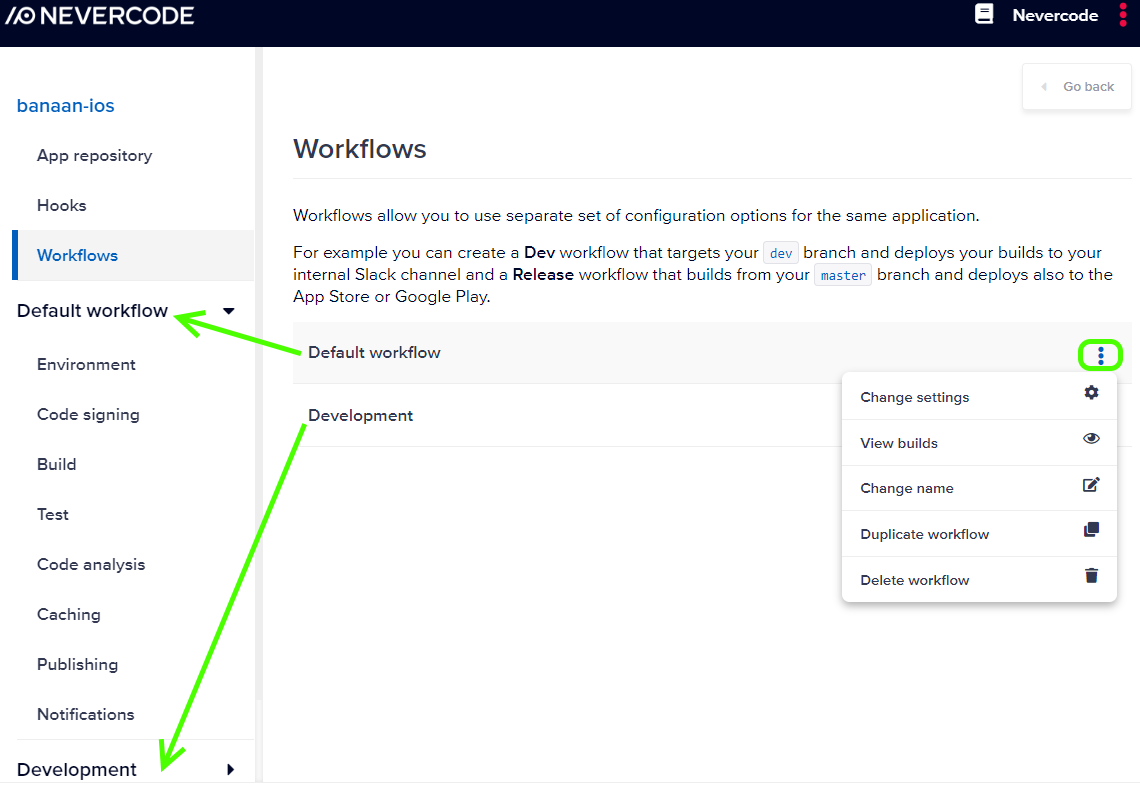In the image, there is a detailed interface belonging to a platform named "Never Code." At the very top, the word "Never Code" is prominently displayed in white within a black bar. This name appears repeatedly, creating a branded header.

The main section of the page is titled "Workflows," which describes how different sets of configuration options can be used for the same application. Specifically, the text explains that you can create a development ("dev") workflow targeting a dev branch for deploying builds to an internal Slack channel, and a release workflow that builds from the master branch for deployment to the App Store or Google Play.

Below this, there is a prominently highlighted section labeled "Default Workflow." A green arrow points directly to this section, signifying its importance. To the right of the "Default Workflow" section, there are three dots enclosed by a green-highlighted circle, indicating that this menu has been clicked. The menu reveals several options: "Change Settings," "View Builds," "Change Name," "Duplicate Workflow," and "Delete Workflow."

On the left side under the "Default Workflow" label, there is a list of workflow components: Environment, Code Signing, Build, Test, Code Analysis, Caching, Publishing, and Notifications. Additionally, there is a separate section or tab for "Development" visible as well.

Overall, the interface is organized to facilitate different workflows for application development and deployment, with a clear emphasis on customization and control over different stages of the development process.